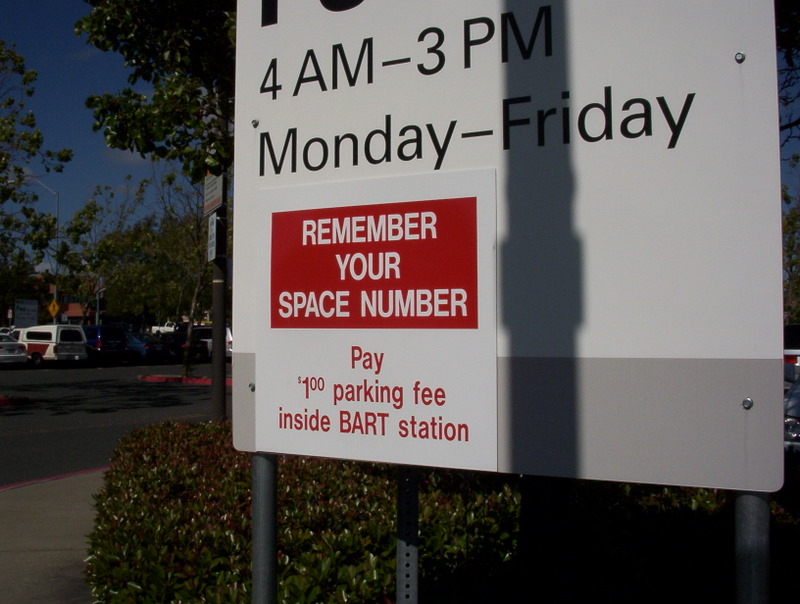The image captures a detailed scene of a parking sign situated alongside a manicured sidewalk. The main sign, mounted on a gray steel pole, features a light gray rectangular board stating, "4 a.m. - 3 p.m. Monday - Friday," indicative of parking regulations. Attached to this is a smaller white sign with bold red and white lettering that instructs, "Remember your space number," and "Pay $1 parking fee inside BART station." Surrounding the sign are trimmed and lush green bushes and trees, evidencing a warm season with their fully bloomed green leaves. In the background, a clear, solid blue sky meets a small parking lot visible to the lower left, showcasing the backs of a few parked cars. The scene is one of organization and clarity, emphasizing the utility and clear instructions of the signs amidst a vibrant outdoor setting.